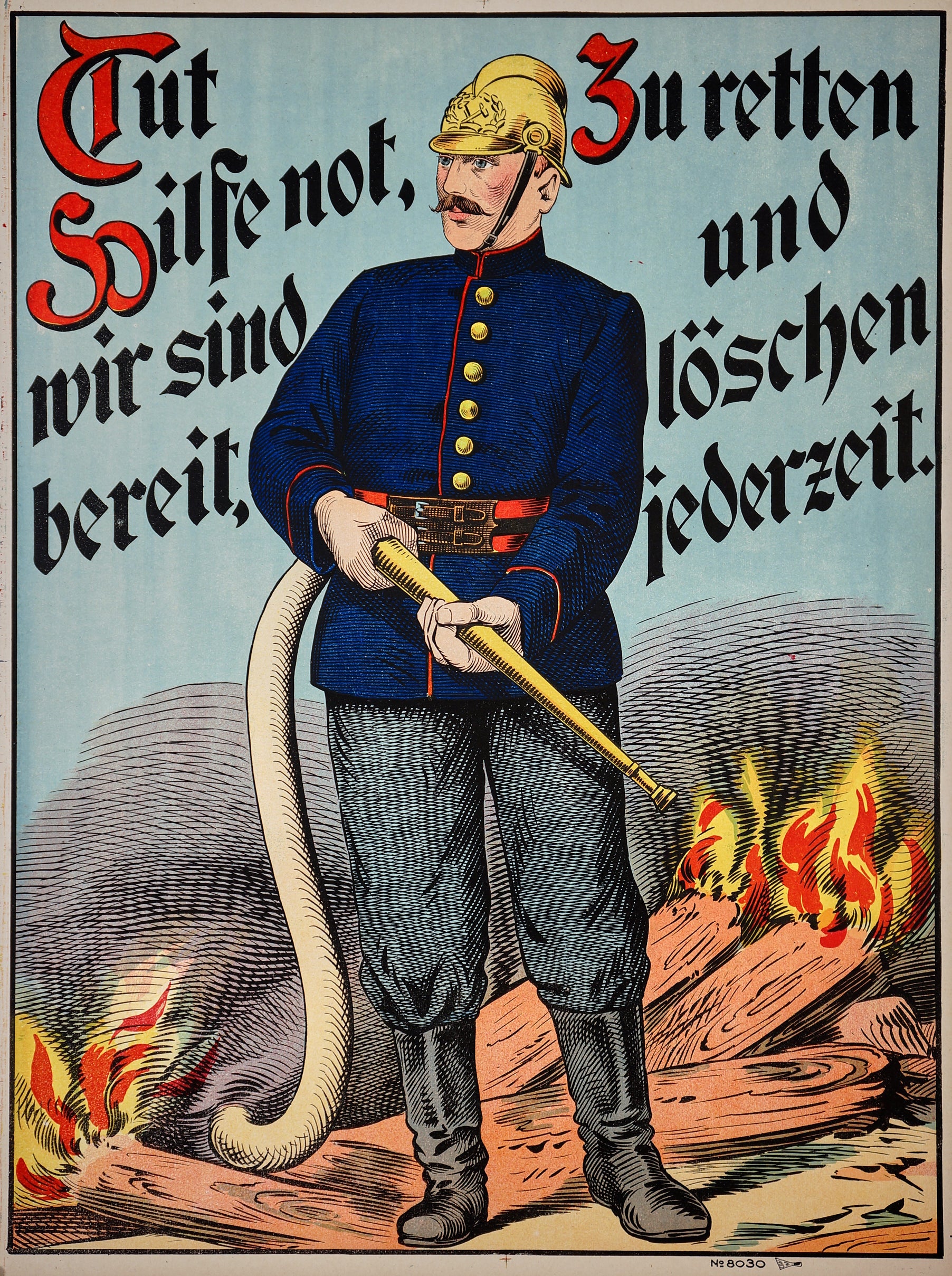This detailed illustration, likely from an old magazine or poster, depicts a 19th-century European firefighter, possibly from Germany. The firefighter, drawn with inky hatch lines, wears a gold helmet with a prominent, ornate design and a chin strap. He sports a handlebar mustache and is clad in a royal blue jacket with seven gold buttons and red trim around the belt, shirt, and sleeves. His attire includes black pants tucked into black boots. The firefighter holds a vintage fire hose, its back end a thick white hose, and the nozzle is slender and golden. The background features wooden planks engulfed in flames, producing gray smoke that drifts into a blue sky. Additionally, there is German script in ornate, italicized lettering across the top that reads "Toot Swipe or not. There's inspirite to retin and Lucien Yadir tight," with the initial letters in red.